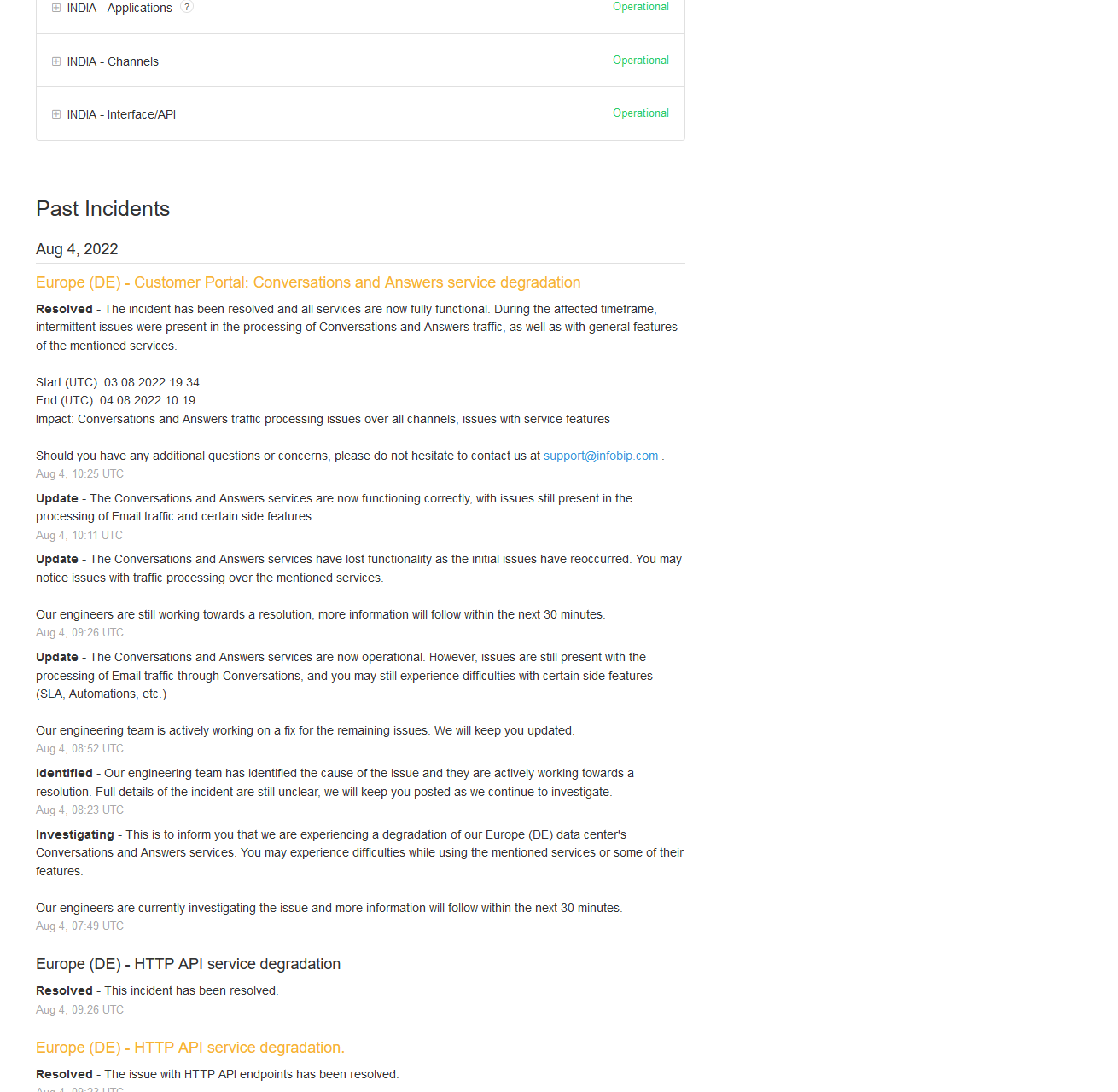This image appears to be a screenshot of a status dashboard or incident report. At the top of the image, there is a section that indicates the current operational status of different India-based services. These are:

- India Application: Operational
- India Channels: Operational
- India Interface: Operational
- API Operational

Beneath this, the image details a past incident from August 4, 2022, specifically relating to Europe (DE) Customer Portal. The incident affected the Conversations and Answers services, resulting in service degradation. The issue has since been resolved, and it is indicated that all services are now fully functional. However, during the affected time frame, further complications were noted. 

It is mentioned that despite the resolution of the primary incident and the restoration of Conversations and Answers services, there were ongoing issues related to the email traffic and certain side features. Additionally, there is a reference to the functionality of Conversations and Answers services being compromised during the incident, mentioning a reoccurrence of issues, though the specific details remain unclear due to the poor quality of the image.

Overall, the screenshot communicates the operational status of various services, the nature and resolution of a past incident, and lingering issues that were encountered.